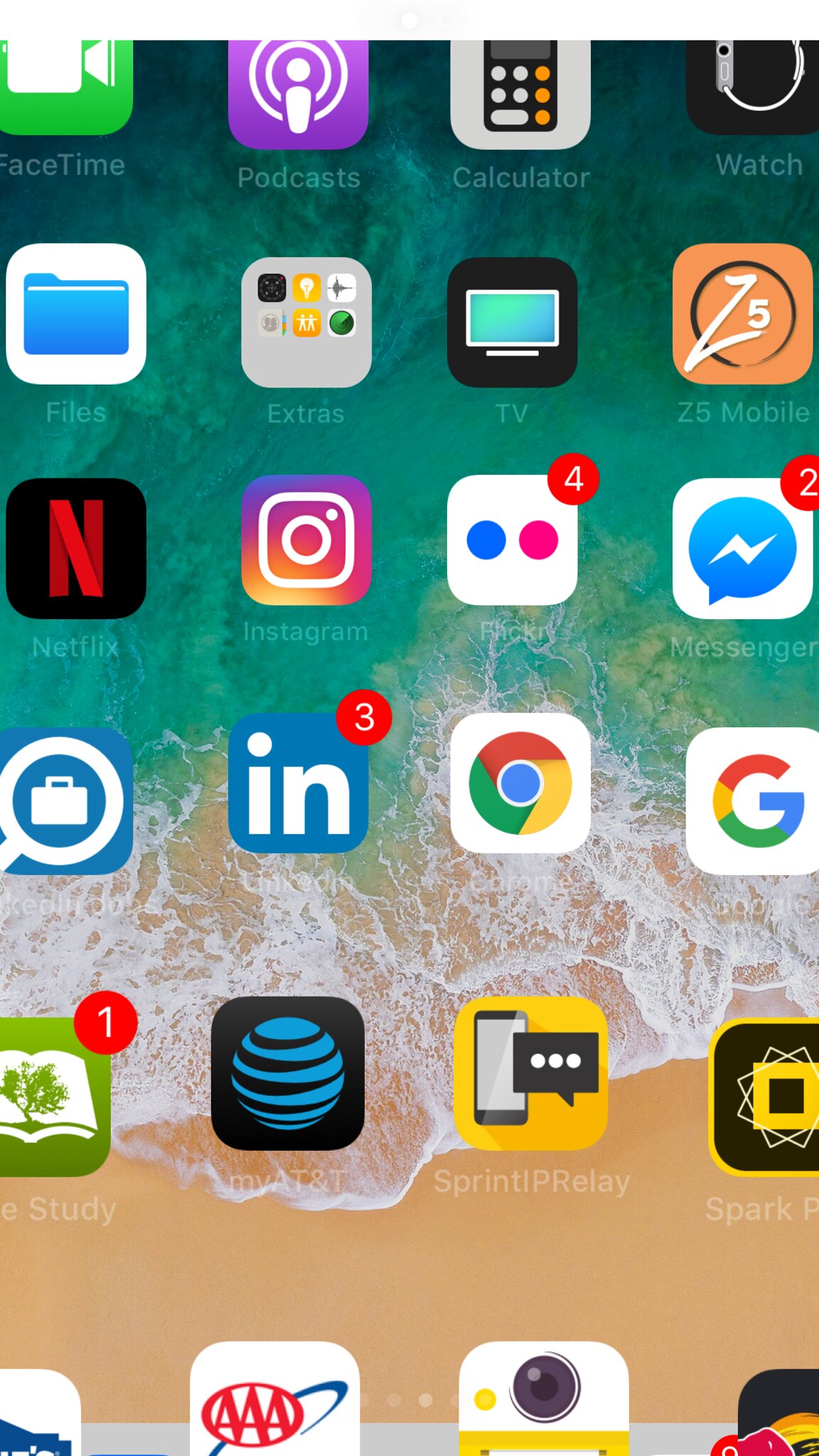This image is a close-up screenshot of a portion of a smartphone (likely an iPhone) home screen showing a grid of app icons arranged in four columns and six rows. The icons belong to various commonly used apps like Messenger, Google Chrome, LinkedIn, Google Files, Video Calculator, and Apple Watch, each with distinct colors and designs. The background of this screen is a serene, lightly saturated image of ocean waves gently washing onto a sandy beach. Below each app icon is a label with very pale text, making it somewhat difficult to notice at first glance. There are also notification markers on several app icons: four on Flickr, two on Messenger, three on LinkedIn, and one on another app related to studying.